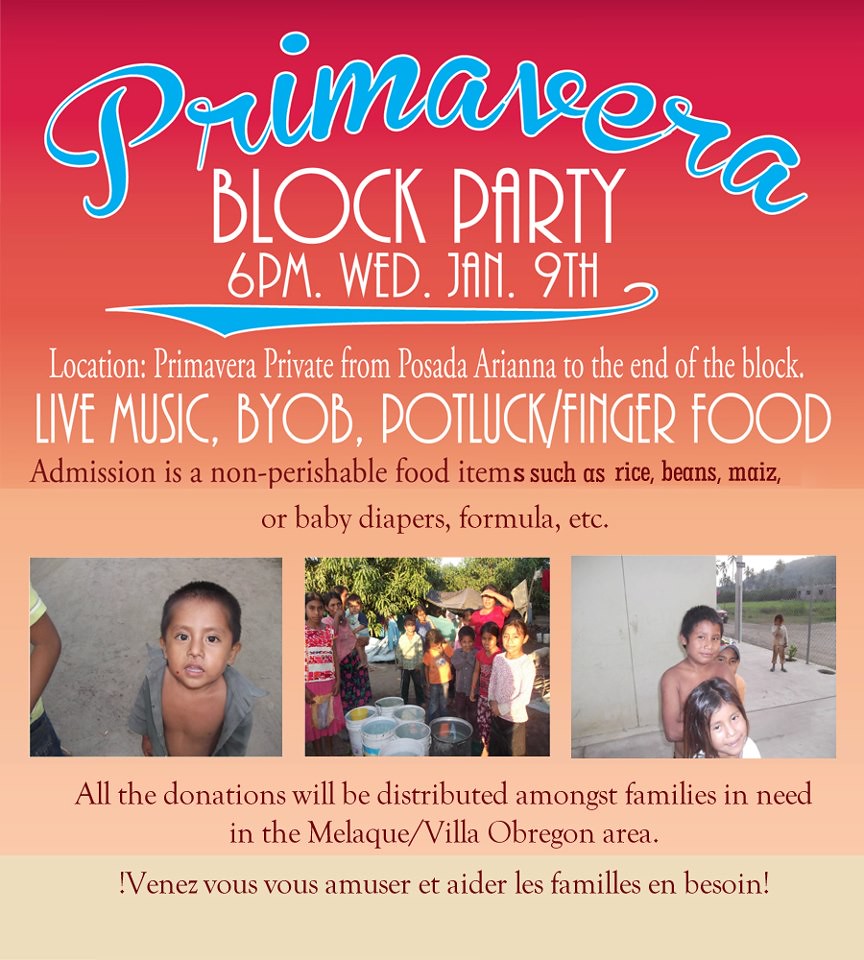Advertisement poster for a community block party with a colorful red-to-white gradient background. A prominent headline in blue cursive reads "Primavera," followed by "Block Party" in white font. Event details include "6pm, Wednesday, January 9th," with a decorative blue underline. The location is specified as Primavera, private from Posada, Ariana, to the end of the block. Activities will feature live music, BYOB, and potluck finger food. Admission requires a non-perishable food item donation such as rice, beans, maize, baby diapers, formula, etc., with all donations benefiting families in need in the Merlakey/Villa Obregon area. Below this, three photographs depict children of Hispanic descent: one showing kids playing outside, another with children around buckets, and a third with a little boy with an open shirt. A Spanish sentence expresses that the event is for fun and aid for families in need.